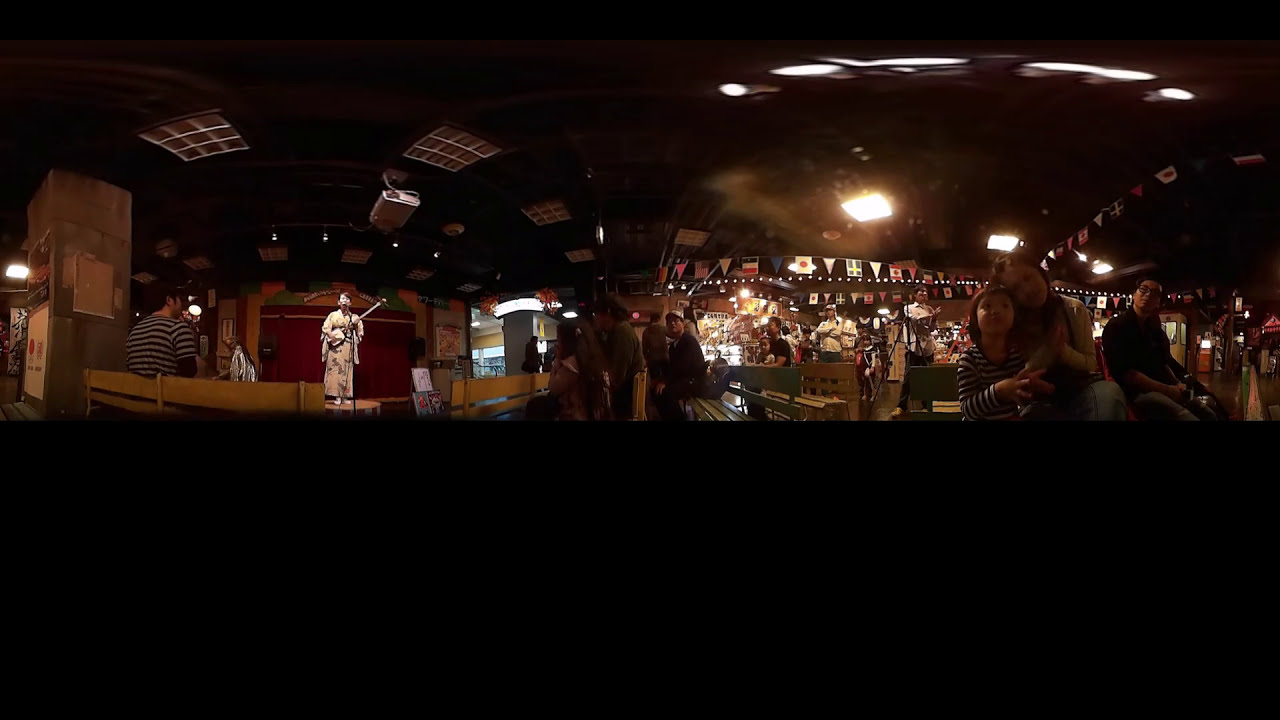The panoramic image captures an indoor venue, likely resembling an international bar or restaurant, featuring a performance on a small stage. On the left side of the stage, dressed in a kimono, stands a woman playing a traditional Japanese string instrument against a backdrop of a red curtain. In the left foreground, a man in a black and gray striped shirt and cap sits on a bench, engrossed in the performance. The scene unfolds to the right, revealing more rows of benches filled with an audience of around ten people, with additional onlookers standing behind the seating area. The setting exudes an international ambiance, as indicated by strings of various national flags draped along the wall. On the far right of the image, a woman tenderly hugs a child, and a man with his head tilted slightly clockwise observes the performance. The room is dimly lit except for focused stage lights, and features a black ceiling dotted with fixtures, including a projector on the left side. The 360-degree view offers a comprehensive glimpse into the intimate atmosphere of the venue.